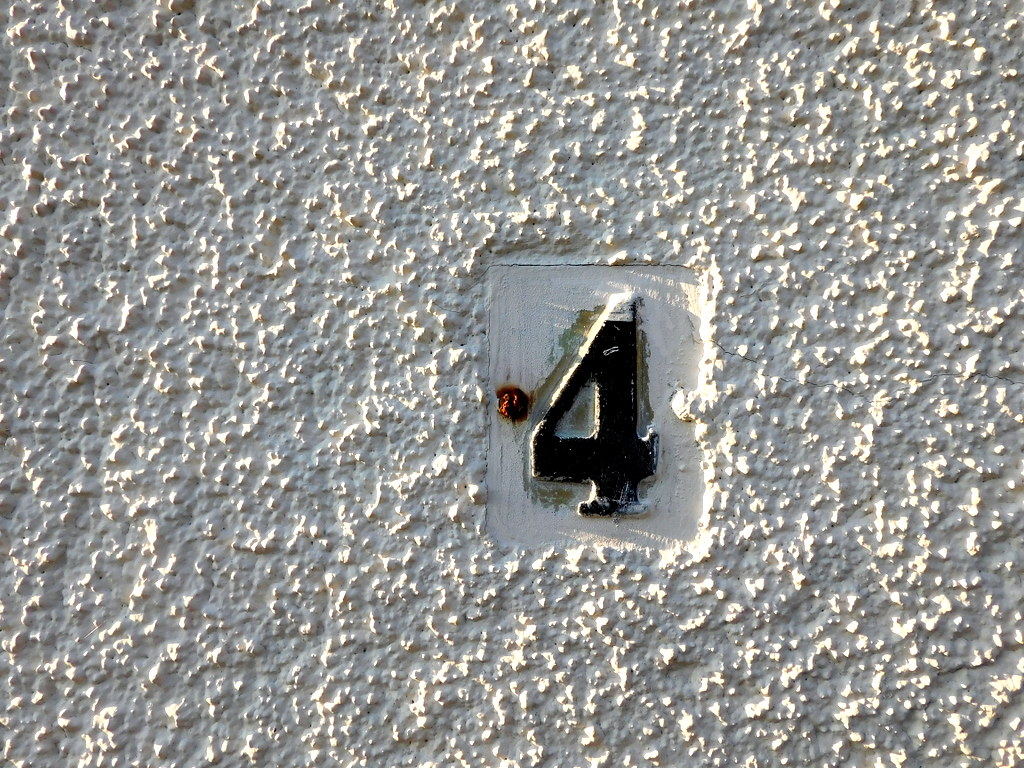The image depicts a rough cast or stucco wall, likely part of a dwelling, with the number "4" prominently displayed in the center on a white rectangular plate. The number "4" is painted in bold black and exhibits signs of wear, including scratches and slight paint misalignment that reveals the original color beneath. The plate is attached to the wall with two screws; the left screw is heavily rusted, making its removal nearly impossible, while the right screw is painted white and largely blends into the background. The sunlight shining on the speckled, granular wall accentuates its texture, adding to the vintage appearance of the overall scene.